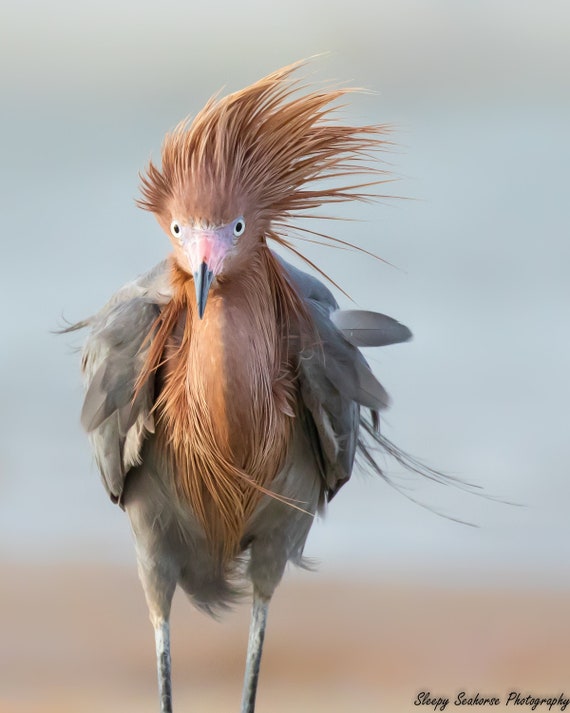In this up-close photograph taken by Sleeping Seek Horse Photography, an unusual bird stands prominently in the foreground against a very out-of-focus, grayish background that might represent a cloudy sky or possibly misty water, tinged with hints of red. The bird has a striking appearance with a blend of colors and textures. Its head features a spiked, feathery crest of brown with wispy feathers that appear windblown, suggesting a breezy day. The bird's face is highlighted by a distinctive black beak transitioning into a pink area near the nostrils, encircled by a patch of white. Its eyes are captivating with large black pupils set against solid white, giving a sharp and focused gaze. The body showcases a mix of orange and gray feathers; the orange covers the crest, head, and breast, while its sides and bottom are adorned with gray feathers that appear slightly ruffled. Its slender, gray legs, about two to three inches long, support the bird as it stands in what looks like a field of brown. The unique combination of features and the dynamic presentation make this bird a striking subject in the photograph.